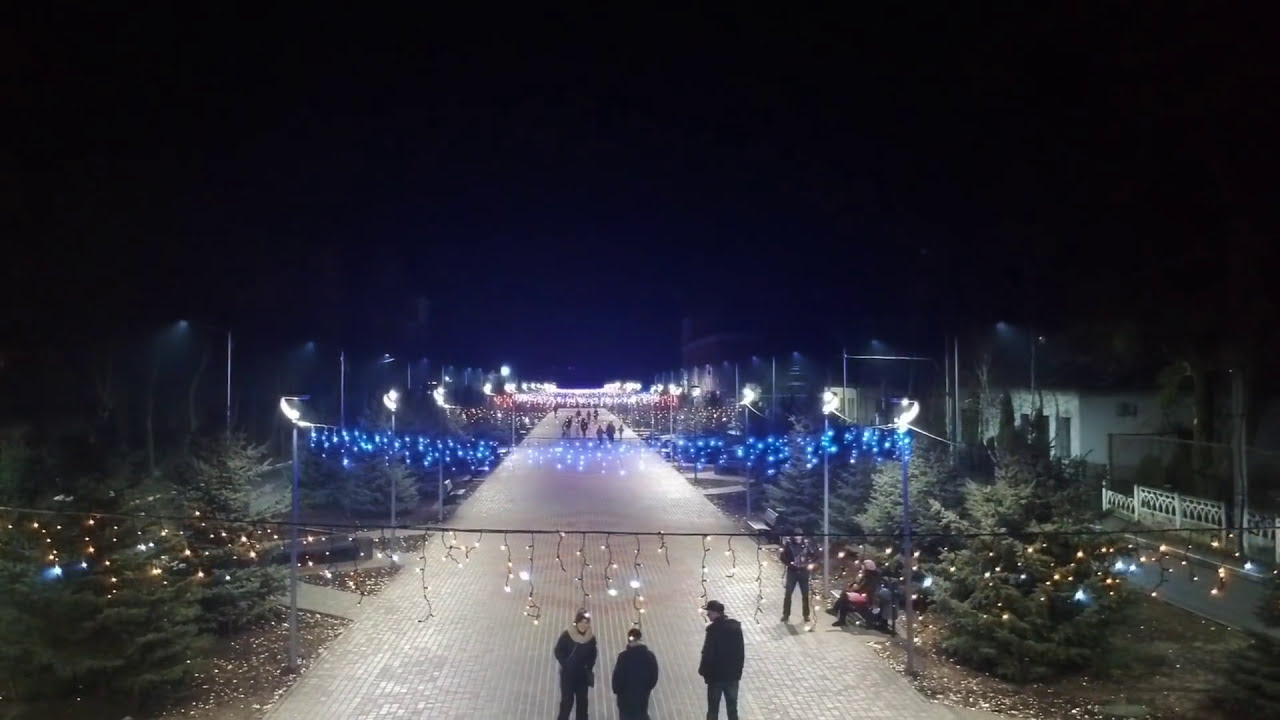This detailed, nighttime, aerial photograph captures a bustling Christmas tree farm or winter display, viewed from above. The scene is illuminated by a series of festive holiday lights strung between poles on either side of a broad, white pathway, which converges into the distance at the center of the image. Rows of lights in variations of white, blue, yellow, and red hang overhead, enhancing the artificial glow that pierces the dark blue and black sky. The pathway is flanked by large, dark green pine and balsam trees, imbuing the scene with a classic holiday atmosphere despite the absence of lights on the trees themselves. Below the lights, people bundled in coats navigate the pathway, with a group of three men standing in a semicircle, engaged in conversation near the foreground. On the right side of the image, spotlights project downward, revealing a few buildings, including a house and a gate, partially cloaked in shadow. The colors in the composition range from black, white, gray, and blue to yellow, green, tan, and brown, creating a vivid and realistic representation of a winter night at a festive outdoor setting.